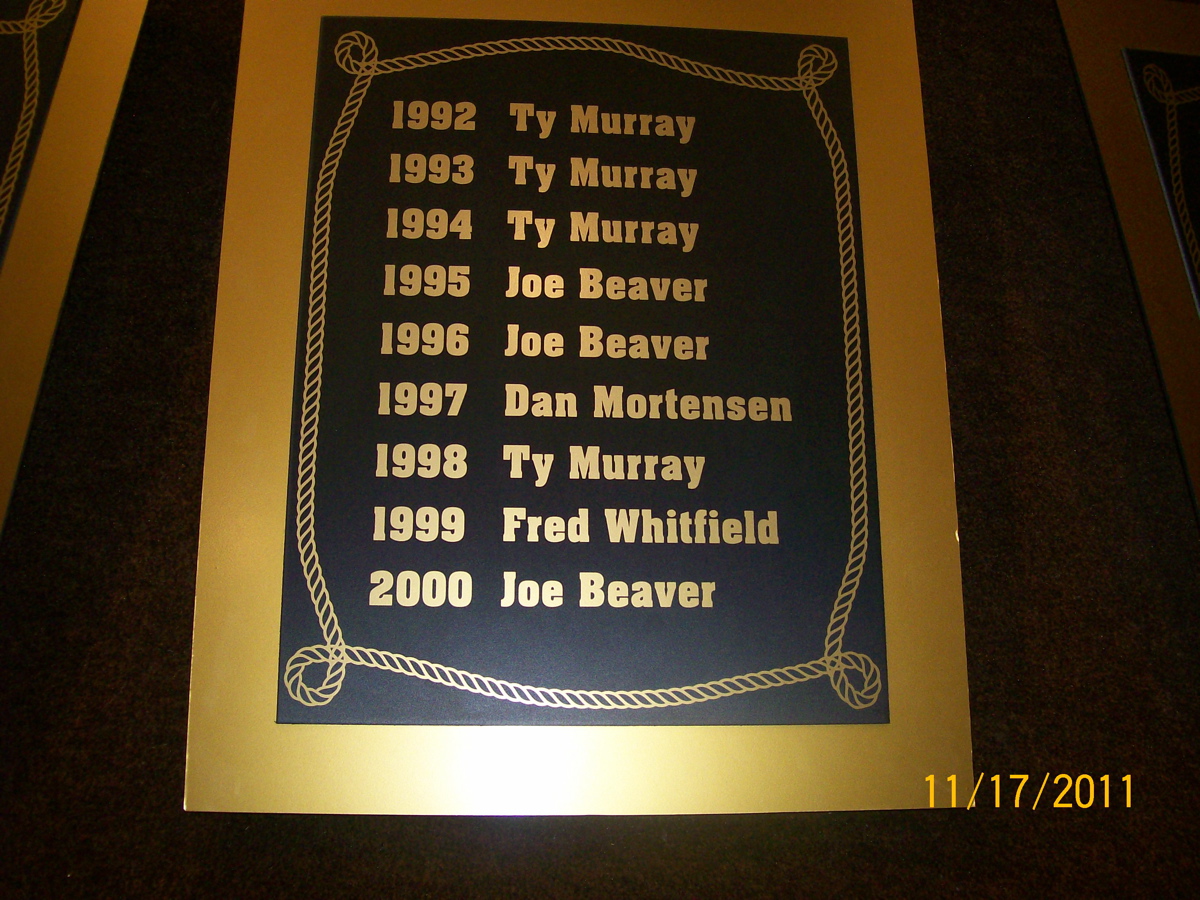The image depicts a gold rectangular plaque mounted against a wooden backdrop. The plaque features an intricate gold perimeter with an inner gold rope design framing the text in the center. The text lists competition winners from 1992 to 2000 in gold lettering on a very dark brown, almost black, background. The names and years are inscribed as follows: Ty Murray for 1992, 1993, 1994, and 1998; Joe Beaver for 1995, 1996, and 2000; Dan Mortensen for 1997; and Fred Whitfield for 1999. In the bottom right corner, there is an imprint dated 11-17-2011.